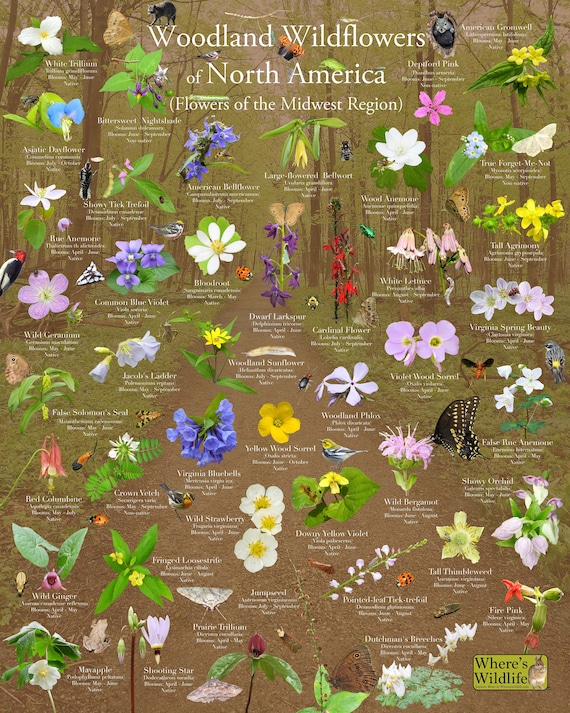This detailed, earthy-toned poster titled "Woodland Wildflowers of North America" features a comprehensive guide to the wildflowers native to the Midwest region. Adorned with lush shades of tan and greenish-tan, the poster showcases small, delicate illustrations of approximately 30 to 50 different wildflowers, each paired with their characteristic foliage. The vibrant flowers, predominantly pink, white, and yellow, are reminiscent of a rainbow, capturing the diversity one might find in a wildflower garden. Accompanying each flower illustration are two lines of text: the traditional English name and possibly the Latin name, followed by an indiscernible minuscule description in white lettering.

The background of the poster resembles a tranquil forest path, with brown earth winding through verdant grass, mold, ferns, and upright trees, creating a serene natural setting. At the bottom right corner, a green square features dark green lettering that reads "Where's Wildlife?" with an image of a rabbit, adding a whimsical touch to the informative layout. The simplicity and muted elegance of the flower illustrations, set against the serene forest backdrop, make this poster both an educational and visually pleasing depiction of woodland wildflowers.